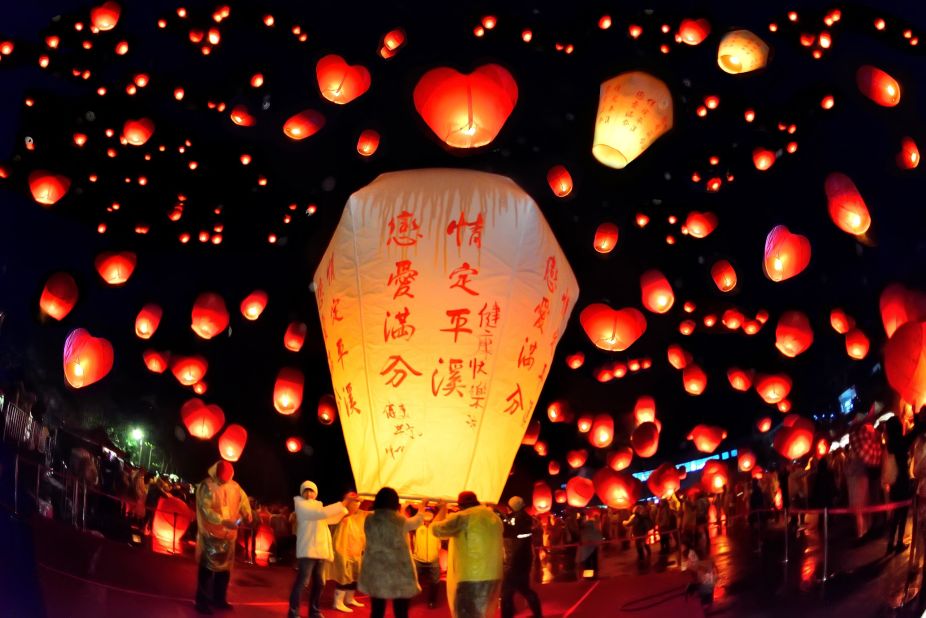In this evocative nighttime scene set against a pitch-black sky, a massive lantern adorned with prominent red Chinese characters takes center stage. The lantern, glowing brightly with a yellow hue at its base where the flame resides, is held at eye level by four to five individuals. These people, dressed in a mix of clean, unique shirts and varied outerwear including coats, hats, and raincoats, form a protective semicircle around the lantern. They're poised beneath it, their figures silhouetted against the candle-lit ambiance. Surrounding this central spectacle, countless smaller paper lanterns, glowing yellow from their internal flames and tinged red around the edges, ascend gracefully into the night sky. The entire scene, imbued with vibrant red and yellow hues, is reminiscent of a celebratory event, likely an Asian festival such as the Chinese New Year. In the foreground, faintly visible under the soft glow of purple and violet ground lights, a metal guardrail and its stands mark the perimeter of this mesmerizing gathering. The atmosphere is further accentuated by the quiet energy of people releasing and gazing up at these floating illuminations, their faces lit by the soft, dancing lights overhead.